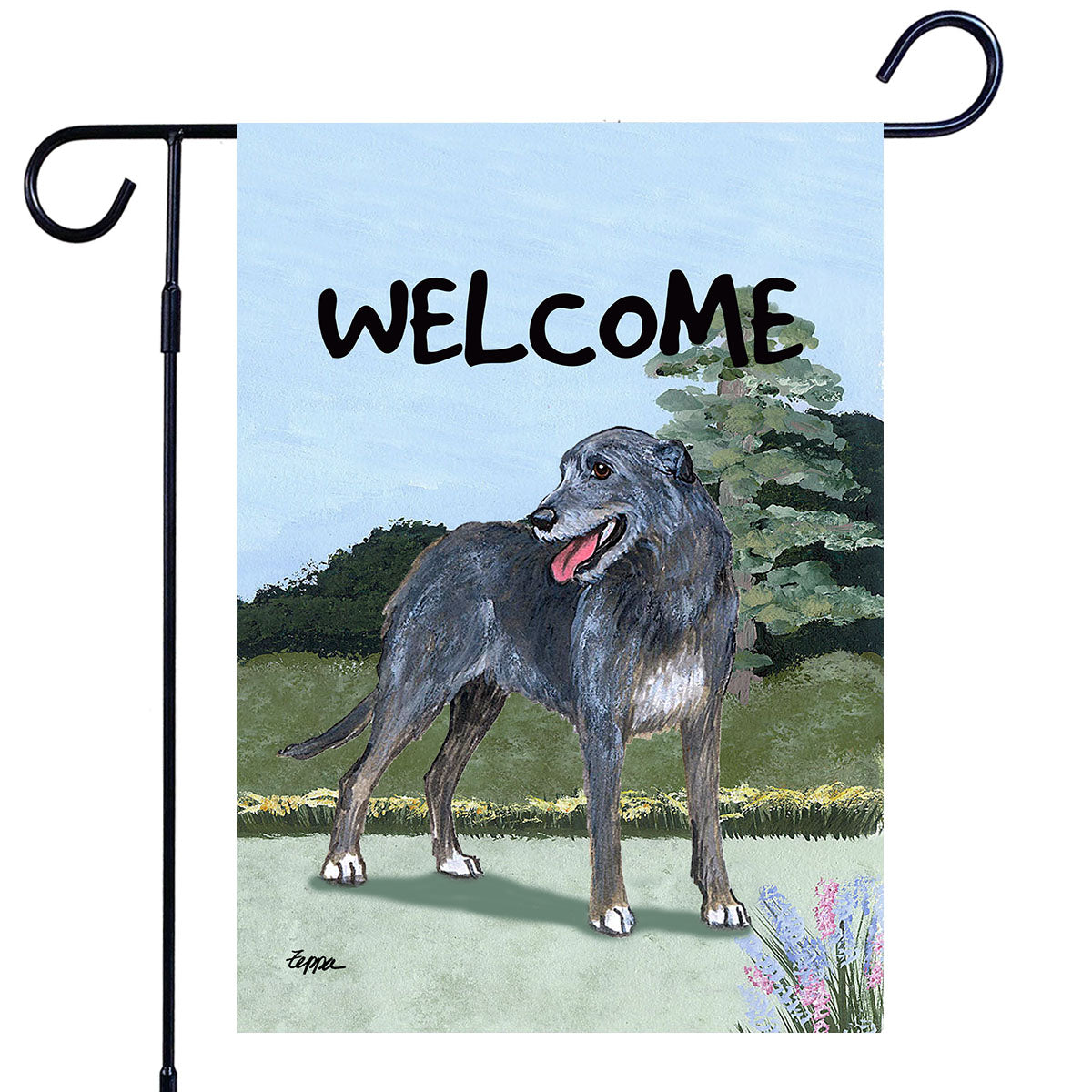This image depicts a garden-sized flag hanging from a black metal frame, typically used as a lawn or garden banner. The flag showcases the word "Welcome" written in a hand-drawn black font over a background that appears to be a print of an acrylic painting, featuring a happy, shaggy gray dog, akin to an Irish wolfhound. The dog, with big brown eyes, a bluish-gray coat, and a bit of white on its chest, stands on a sidewalk surrounded by a green field, with grass, plants, and muted trees and bushes in the background. Pink flowers add a touch of color to the scene, primarily in the right corner of the flag. The overall artwork has a waterpainted effect, characterized by its soft, muted color palette. At the bottom of the flag, "Felipe" is written in cursive, adding a personalized touch to the charming and warmly welcoming design.